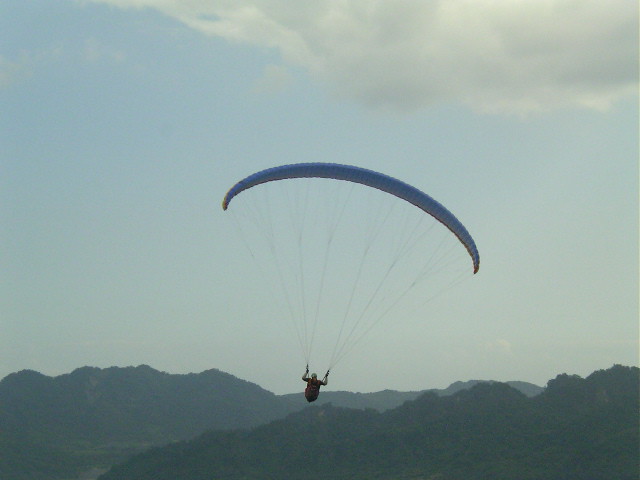In the photograph, a person is parasailing high above a dramatic landscape, their back turned towards the camera. They are gripping a series of almost transparent grey strings that keep them tethered to a large, blue parachute-style canopy, which features red tips. The person, dressed in all dark clothing and strapped into black harnesses, also wears a helmet that appears to be white or grey, offering a hint of safety in this thrilling endeavor. Above the canopy, a solitary white cloud floats in an otherwise clear blue sky, adding to the sense of freedom and exhilaration conveyed in the image. Below, the rugged mountain ranges create a contrasting backdrop with their black and brown hues in the foreground and a blue haze covering the more distant peaks. The photograph captures the essence of adventure, highlighting both the daring sport of parasailing and the stunning natural beauty surrounding the participant.